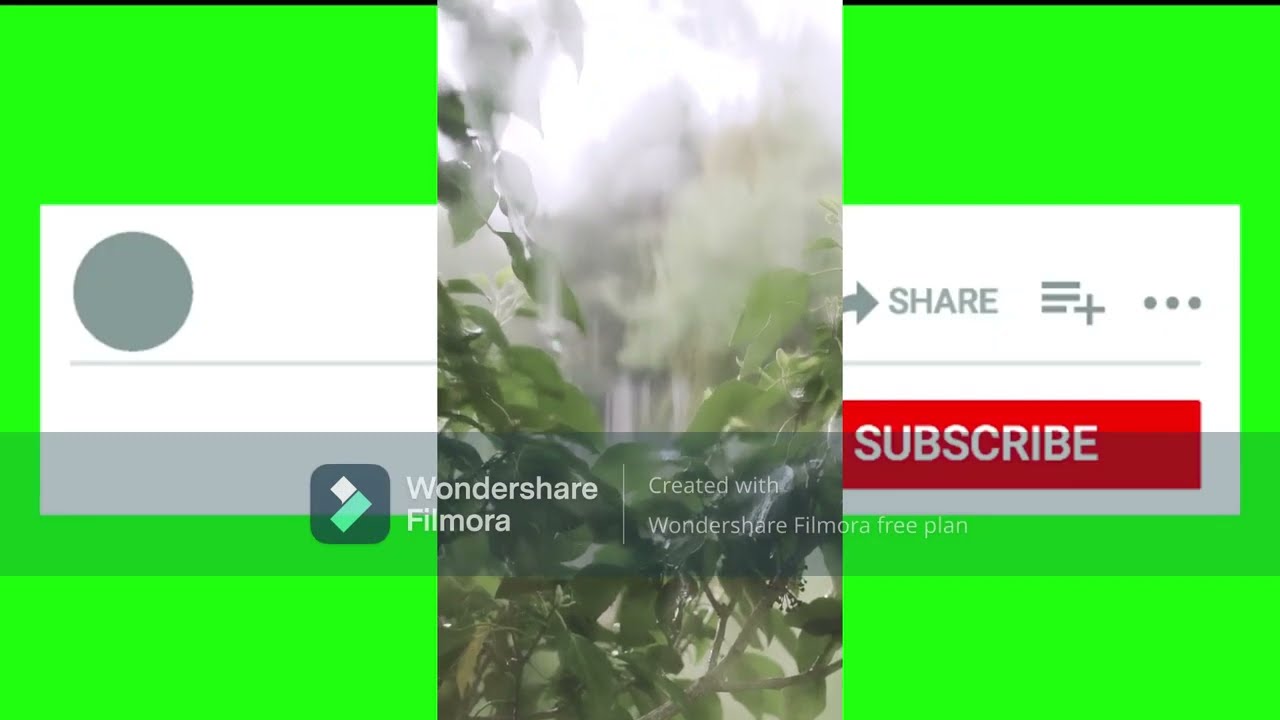The horizontal rectangular image is split into three sections, each framed by a very thin black border at the top that does not extend through the middle section. The left and right sections both feature a lime green background. In the left section, there's a partially visible white and gray rectangular shape cut off by the middle section. This shape includes a gray circle in the top left corner, a gray line underneath, and a gray border at the bottom. Below this shape, the green background transitions into a darker green, and in the lower right corner of this section, there's a gray box containing a white square with a light green rectangle.

The middle section of the image, which is out of focus, displays what seems to be plants and possibly flowers in the foreground, with a blurry white area in the background that could be rocks or more plants. A watermark prominently runs across the lower part of this section, reading "Wondershare Filmora" and "created with Wondershare Filmora Free Plan," with the "W" and "F" extending into the left panel and the latter part of the text spilling into the right panel.

The right section continues the green background and includes the remaining portion of the white rectangular shape from the left section. This part of the rectangle contains the word "Share" with an arrow directed at it, accompanied by horizontal lines, a plus sign, and three dots. Below this is a light gray underline, and at the very bottom, a prominently placed red rectangle with the word "Subscribe" in white letters completes the visual composition.